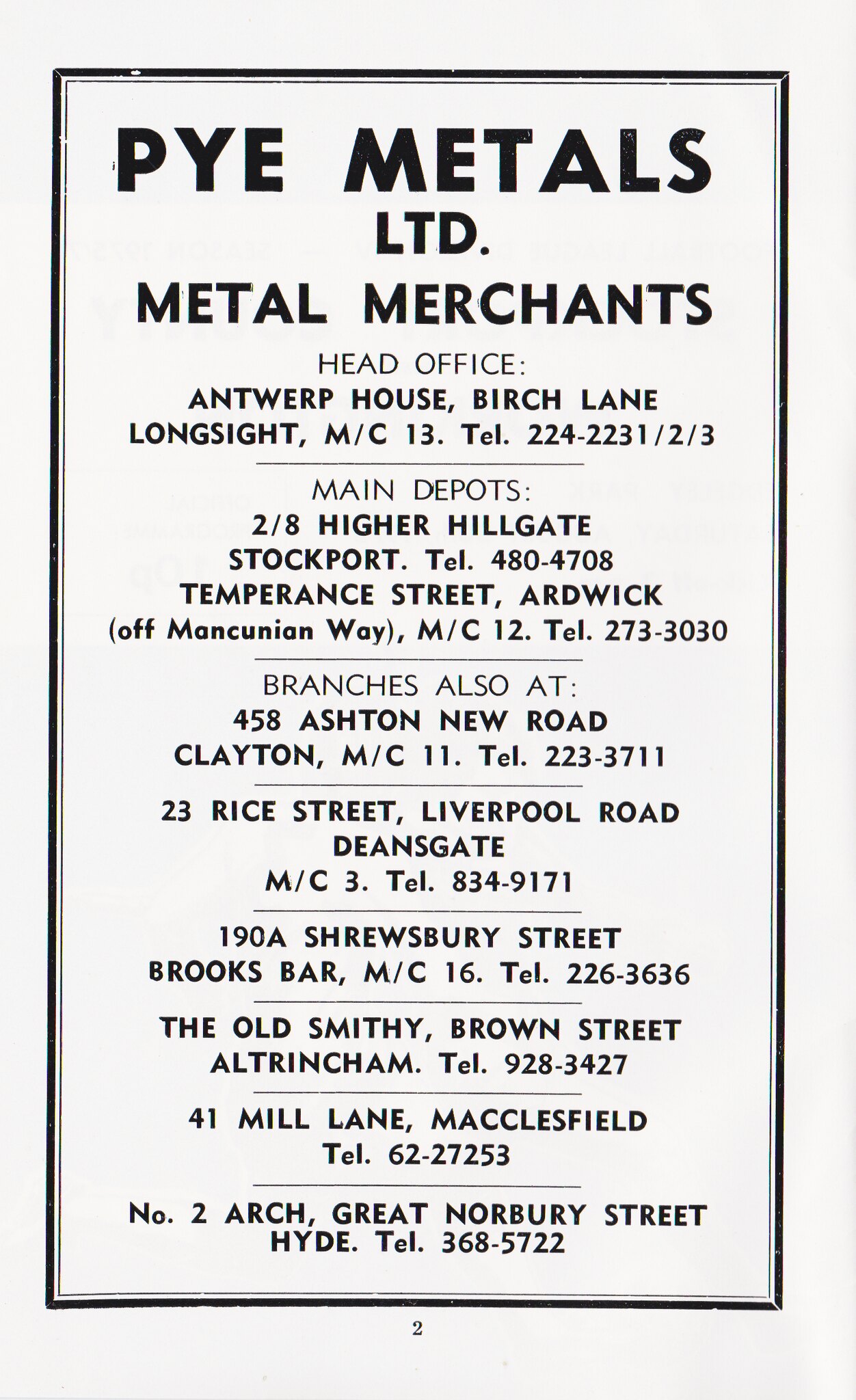This black-and-white flyer for PYE Metals Limited, prominently displayed with a bold black border, presents comprehensive contact information for the metal merchants. The company name, "PYE Metals Limited," is highlighted across the top in black print, followed by the designation "Metal Merchants." The flyer details the Head Office location at Antwerp House, Birch Lane, Longsite, M-Z13, with the telephone number 224-2231-2-3. 

Main depots are listed at 2-8 Higher Hillgate, Stockport, with the phone number 4804708, and at Temperance Street, Hardwick, off Marconian Way, M-C12, reachable at 2733030. Branch locations include 458 Asher New Road, Clayton, M-C11 (phone 223-3711), 23 Rice Street off Liverpool Road, Dean's Gate, 198 Shrewsbury Street (the Old Smith), Brown Street, 41 Mill Lane, Maxley Field, and number 2, Arch Great, Norbury Street. 

The flyer has a vintage aesthetic, complemented by a modern, clean font similar to Helvetica, lending the advertisement an intriguing blend of old and contemporary design elements.